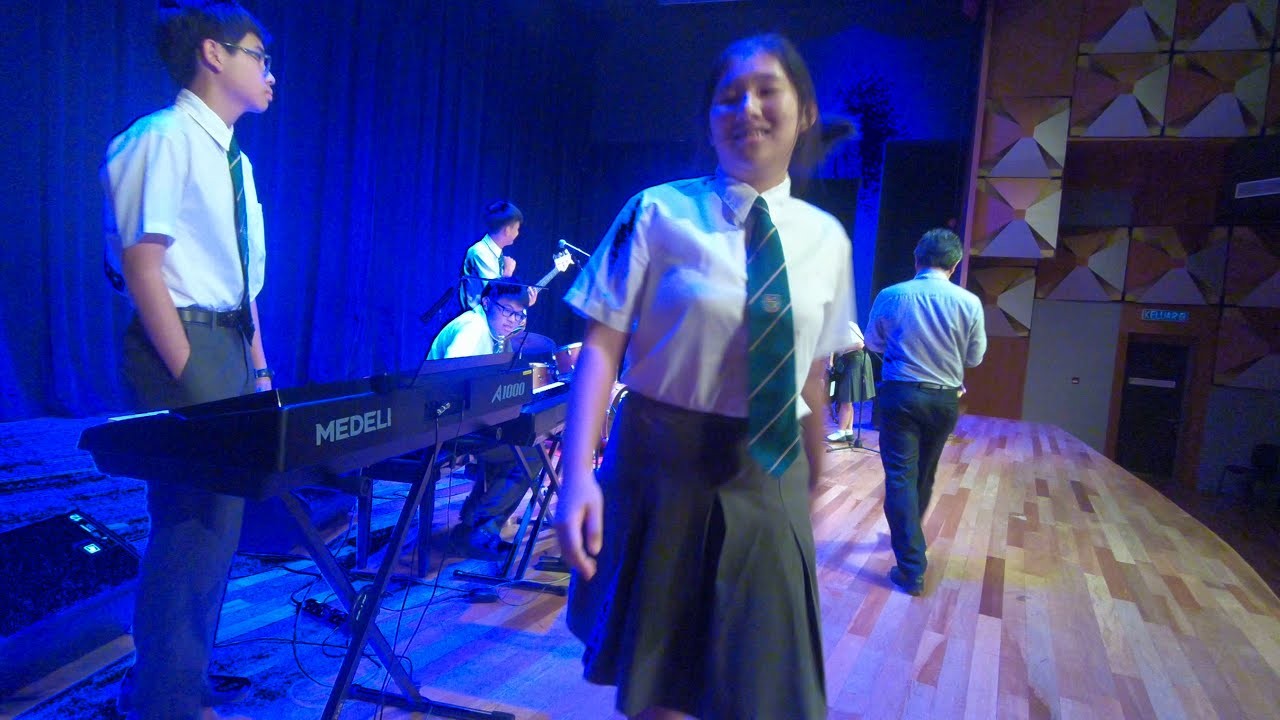The image captures a group of young teenagers dressed in school uniforms, performing or preparing to perform music on a stage. Central to the scene is a smiling girl wearing a white short-sleeved dress shirt, a black skirt, and a green tie, her hair tied in a ponytail, looking directly at the camera. Behind her to the left stands a young man in glasses, hands in his pockets, appearing somewhat disinterested, clad in the same white shirt and tie with dark pants, positioned in front of a keyboard. Further back, another boy is seated at a second keyboard, while to his right, a third boy stands by a drum set with a microphone above him. There is also a young man holding a guitar, situated behind the seated boy. To the right of the smiling girl, a man is seen walking away from the camera, partially obscured. The stage is set in what appears to be a music room or auditorium, with blue curtains adorning the left side and red elements, including a door, visible on the far right where the room gets darker.